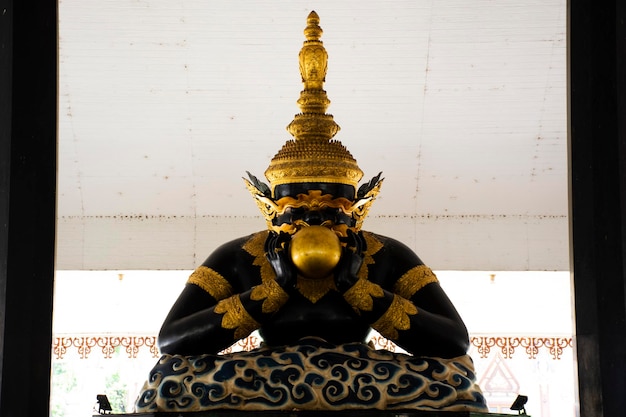This photograph captures a detailed and ornate gold-colored religious statue, likely Southeast Asian and possibly Buddhist, prominently featuring a deity or sacred figure with a symmetrical black and gold body. The statue is seated cross-legged, adorned with numerous golden accessories including a crown that points upward, bracelets, and jewelry around the neck and above the biceps. The figure holds a golden ball with both hands positioned under its chin, giving it a contemplative or forlorn expression. The statue is placed against a white background accented with a reddish pattern, suggesting a shrine or temple setting. It is positioned on a large platform with lights at the base and flanked by black balls, all under a white tent-like or ceiling structure.